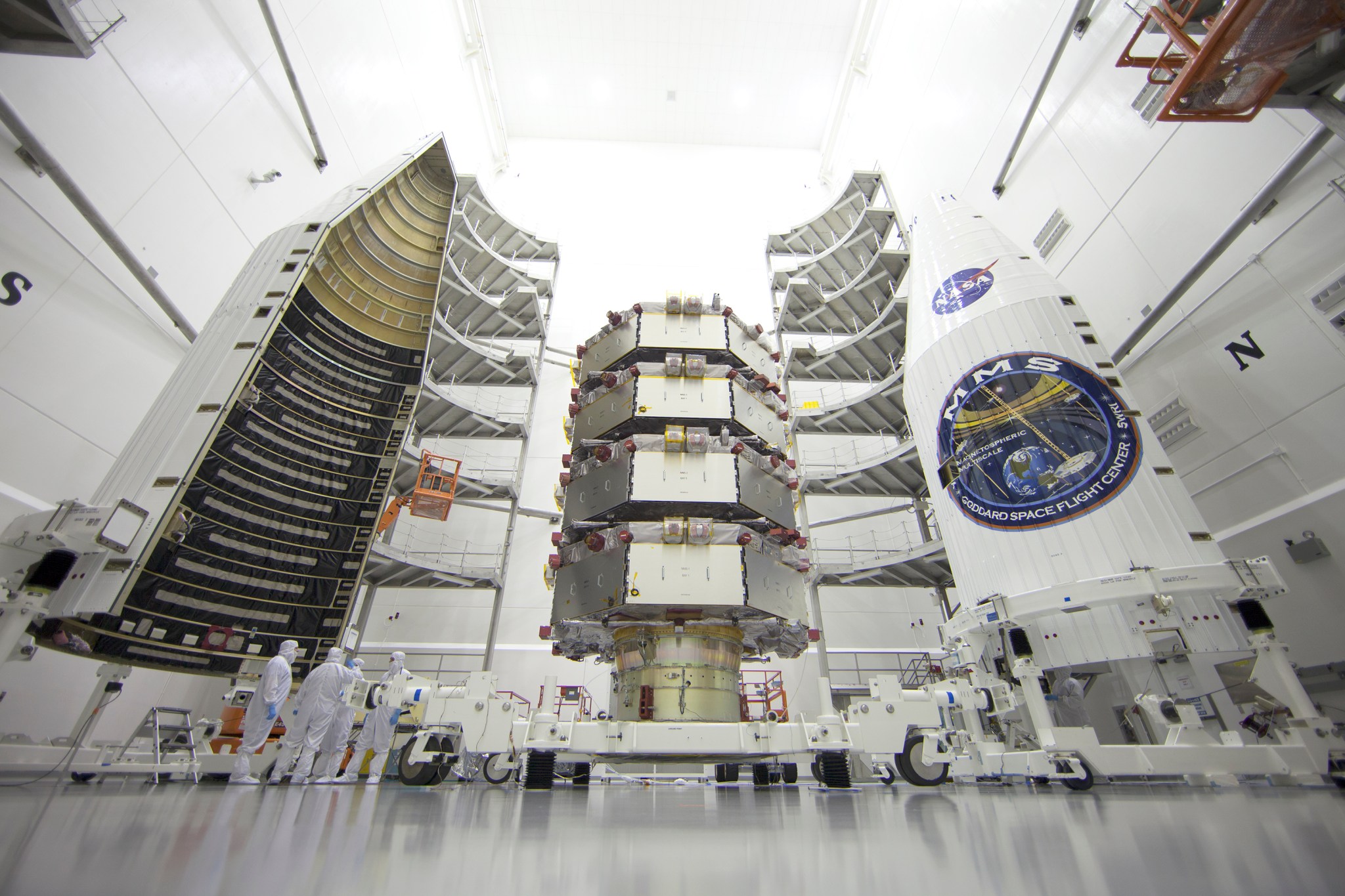In this photograph, we observe an advanced, high-tech laboratory room affiliated with NASA. Prominently displayed in the top right-hand corner is a small space capsule marked with the NASA insignia. Below it, a large emblem bears the inscription "MMS, Goddard Space Flight Center." To the top left of the image, we see detailed cross-sections of another spacecraft or scientific apparatus, illustrating the functions of its various components. 

The lab floor is populated by several individuals clad in full protective suits, including body gloves and masks, suggesting a controlled, contamination-free environment. 

At the center of the photograph stands a unique and sophisticated instrument, likely designed for measuring wavelengths or light waves from outer space. Though its exact function is unclear from the image alone, the device features intricate mechanisms and an array of components, boasting a gleaming array of silver and gold trims among other technical elements, highlighting its high-tech nature.